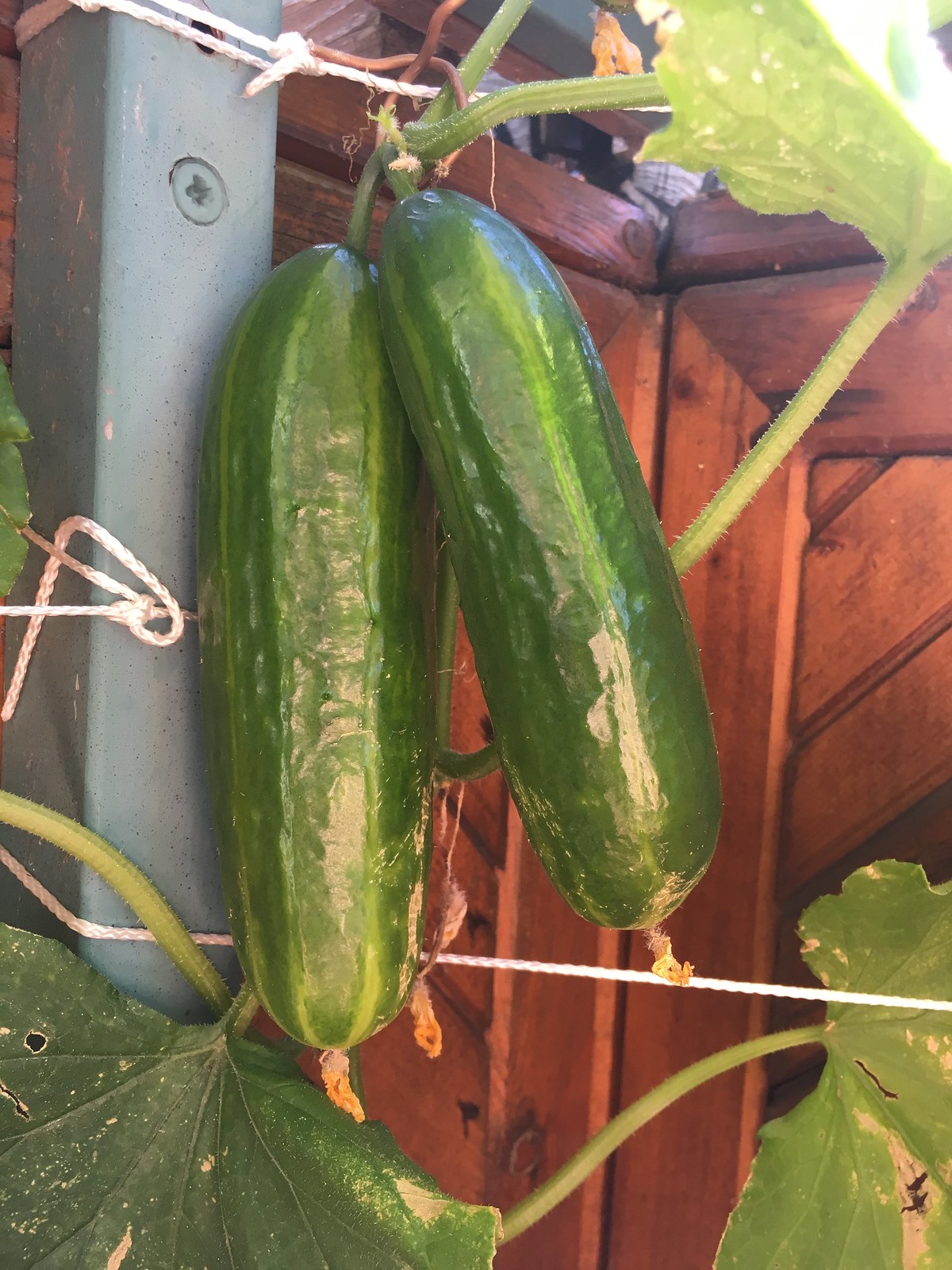In this detailed photo of a backyard garden, a metal pole on the left serves as the primary support structure. A screw is driven into the pole, which holds white string used to support the growth of lush green vines. Two large, cylindrical green fruits—likely either cucumbers or zucchinis—hang prominently in the center of the image. The vines, adorned with a few visible large leaves, are meticulously tied to the metal pole, ensuring the fruits grow properly. The background reveals a wooden enclosure, perhaps part of a fence or a garden boundary, adding a rustic charm. Further back, a glimpse of a house or porch is barely visible, hinting at the garden's residential setting.